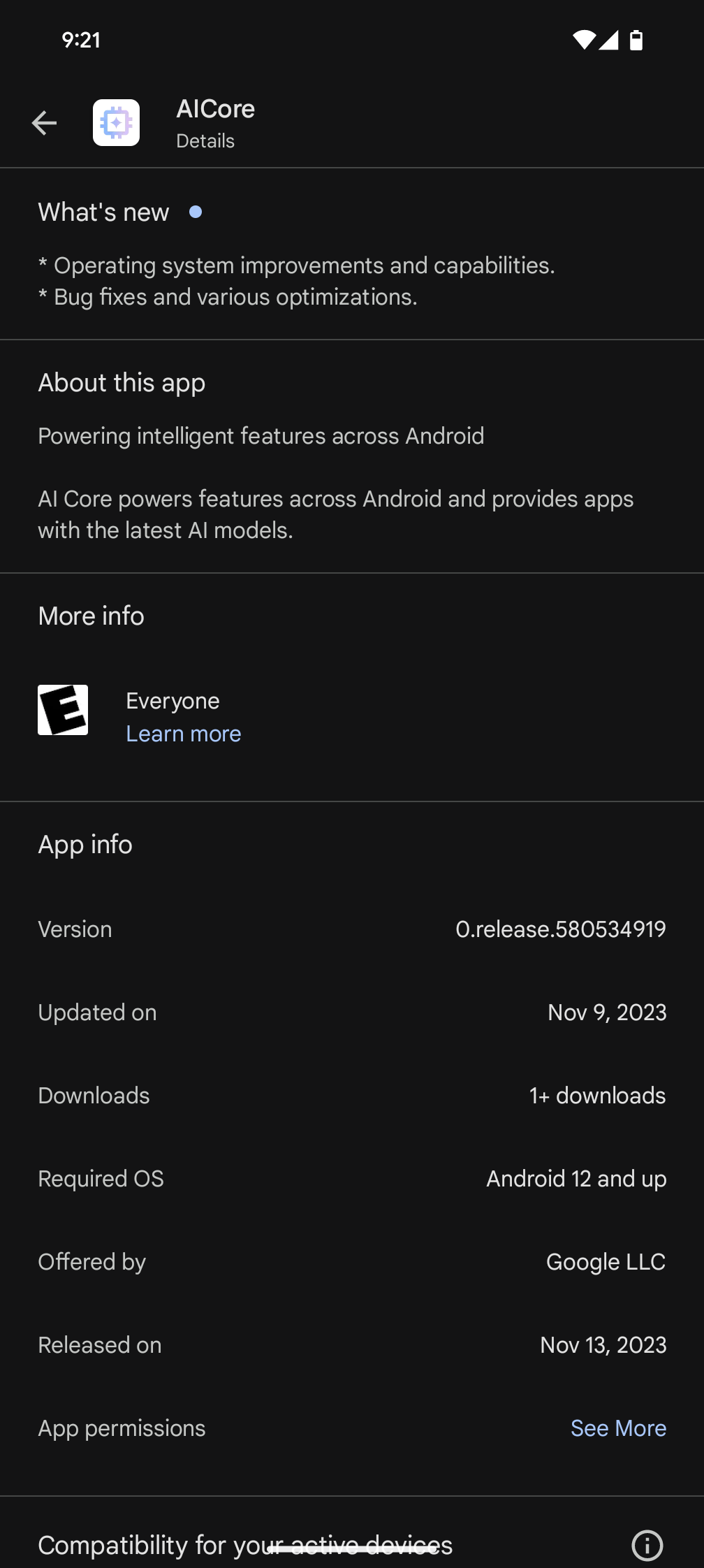**Descriptive Caption:**

The image depicts a detailed application page designed with a smartphone interface. At the very top of the screen, the status bar is displayed against a darker gray or black background, showing the time (9:21) on the left. On the right side of the status bar, icons indicate a full Wi-Fi signal, a full 4G connection, and a battery level at two-thirds.

Moving down, on the top left of the screen, there's a back arrow. Next to it is an icon resembling a small white box with a green chip inside. Adjacent to the icon, in bold white text, reads "AI Core," with smaller white text beneath that says "details." Directly below these elements is a thin white horizontal line spanning the width of the screen.

Underneath this line, there is a header with "What's New" highlighted by a blue dot beside it. The section provides a list of updates including "* Operating system improvements and capabilities," and "Bug fixes and various optimizations."

Continuing downward after another thin white line, in large white text, "About This App" is stated. This is followed by a description in smaller white text: "Powering intelligent features across Android. AI Core powers and features Android and provides apps with the latest AI models."

Further down is a "More Info" section. This includes an "Everyone" rating, with a "Learn More" blue hyperlink underneath. Below this, there is an "App Info" section detailing various information such as version, last update date, number of downloads, required OS, offered by, release date, and operational status.